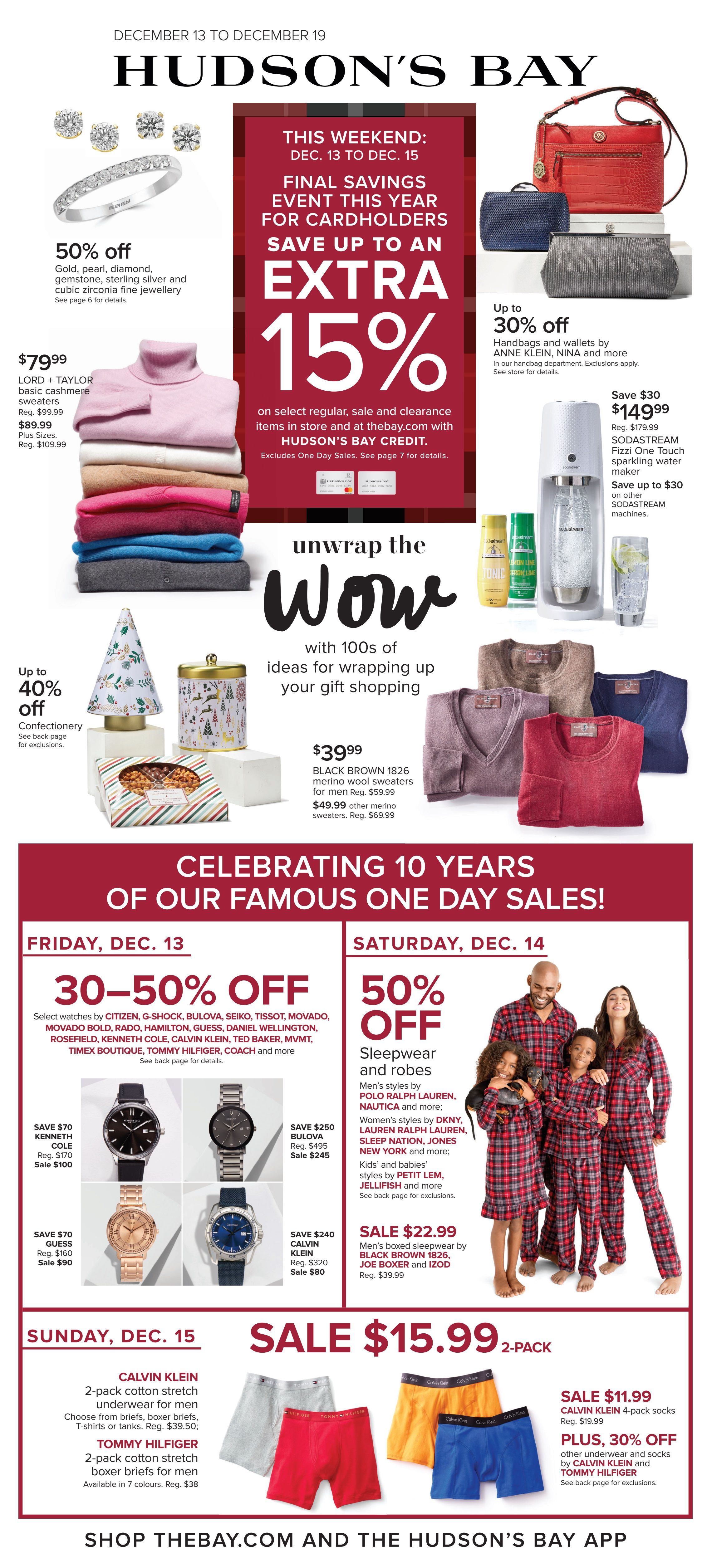Screenshot of a Hudson's Bay Merchandise Sale

The top of the screenshot features the Hudson's Bay logo prominently displayed. Just above the logo, small text indicates the sale period from December 13th to December 19th. Below the name, a vertical red rectangular banner confirms this time frame with white text and highlights an additional 15% discount available for Hudson's Bay cardholders.

Flanking the red banner are various sale items. The top corner features jewelry marked at 30% off, with clothing selections displayed underneath. On the opposite side, the top displays purses and a SodaStream carbonated water dispenser. Below these, decorative accessories and more clothing are showcased.

In the lower half of the image, a squared-off section highlights three distinct sales periods. It kicks off with a red banner proclaiming "Celebrating 10 Years of Our Famous One-Day Sales." The first sale, dated Friday, December 13th, offers 30% to 50% off on watches, featuring four color images with brief descriptions and prices. Adjacent, the second section for Saturday, December 14th, advertises 50% off sleepwear and robes, accompanied by an image of a family wearing matching plaid sleepwear. The third section, for Sunday, December 15th, promotes a sale on undergarments with two-packs priced at $15.99.

At the bottom of the screenshot, information directs customers to shop at shopthebay.com or through the Hudson's Bay app.